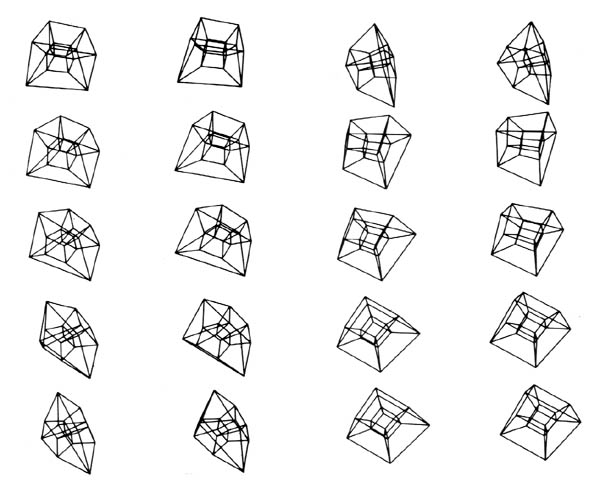This image features an array of 20 unique geometric line drawings arranged in a grid of four rows and five columns on a plain white background. Each drawing depicts a cubicle-like shape rendered in black lines, resembling three-dimensional forms. The shapes vary in appearance, some resembling lopsided rhombuses, diamonds, or squares seen from different perspectives, giving an impression of depth and varying orientations. Despite the uniform line weight, every shape is distinct and none are identical. Some configurations include intricate interior lines, creating the illusion of squares within squares or nested boxes, connecting and intersecting in complex ways, almost appearing like abstract pencil or pen sketches of pyramids or cubes viewed from differing angles.